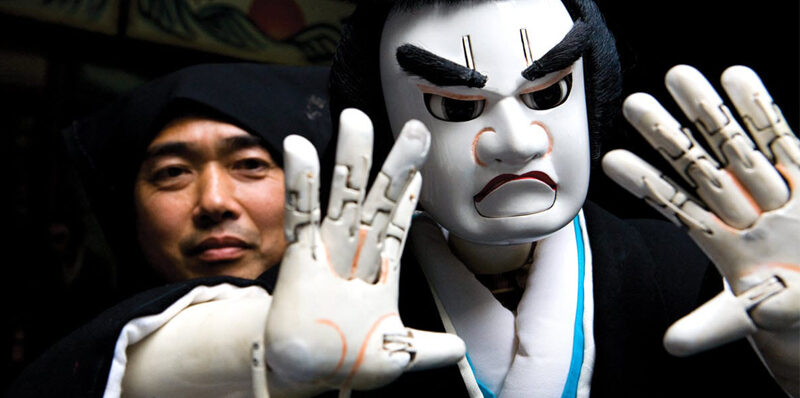The photograph, taken indoors, captures a striking scene dominated by a mechanical puppet and its puppeteer. The rectangular image, approximately six inches wide and two inches high, is framed with a darkened background that focuses attention on the subjects. On the left side, a man of Asian descent is visible, adorned in black clothing and a black hood or beanie that conceals his hair. His gaze is directed slightly to the right, where he is holding an intricately designed puppet.

The puppet, a human-like doll with cream-white skin, commands the majority of the right-hand side of the image. It features large, expressive black eyebrows that are currently furrowed, giving it an unhappy and intense expression. The puppet's eyes are equally large and its hair, made from a thread-like fabric, is also black. The puppet has orange lines accentuating its hands and face, and its articulating joints in its fingers and mouth suggest advanced mechanical design, allowing the puppeteer to imbue it with lifelike motions and varied expressions.

The puppet is dressed in a traditional-looking garment resembling a kimono, featuring a black robe with a white inside collar trimmed in blue. Its white plastic hands are raised, palms facing forward, exposing the detailed articulation of its joints. The man behind the puppet appears to be half-smiling with his eyes, though his mouth remains neutral, adding a subtle complexity to his expression.

Together, the puppeteer and his puppet present a visually captivating tableau, blending traditional cultural elements with modern mechanical artistry in a vividly detailed indoor setting.